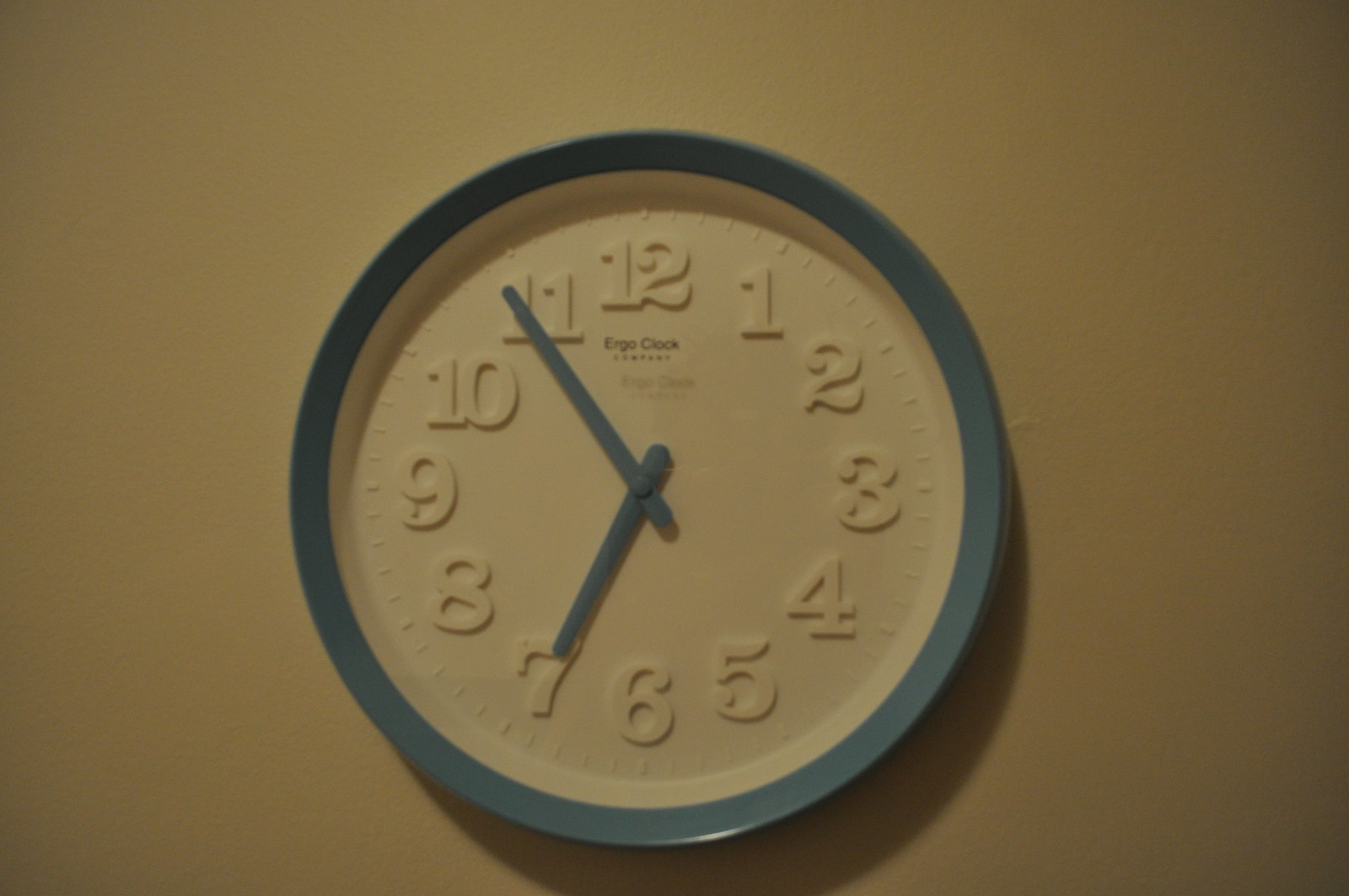The image depicts a round clock mounted on a wall that appears to be a dark yellow. The clock's face is completely white and features white numbers and minute markings in a distinctive, fun font, all of which seem to be slightly raised, reminiscent of Braille text. The clock, which could be mistaken for a beautiful ceramic dinner plate or pie dish, has a striking blue rim that matches the blue hour and minute hands. The minute hand is pointing at the 49-minute mark, just before the 11, while the hour hand is on the 7. Below the 12 on the clock's face, there is black writing that reads "Ergo Clock," and there is additional black text below the 11, though it's not entirely legible. The clock casts a shadow on the wall behind it, adding depth to the scene.